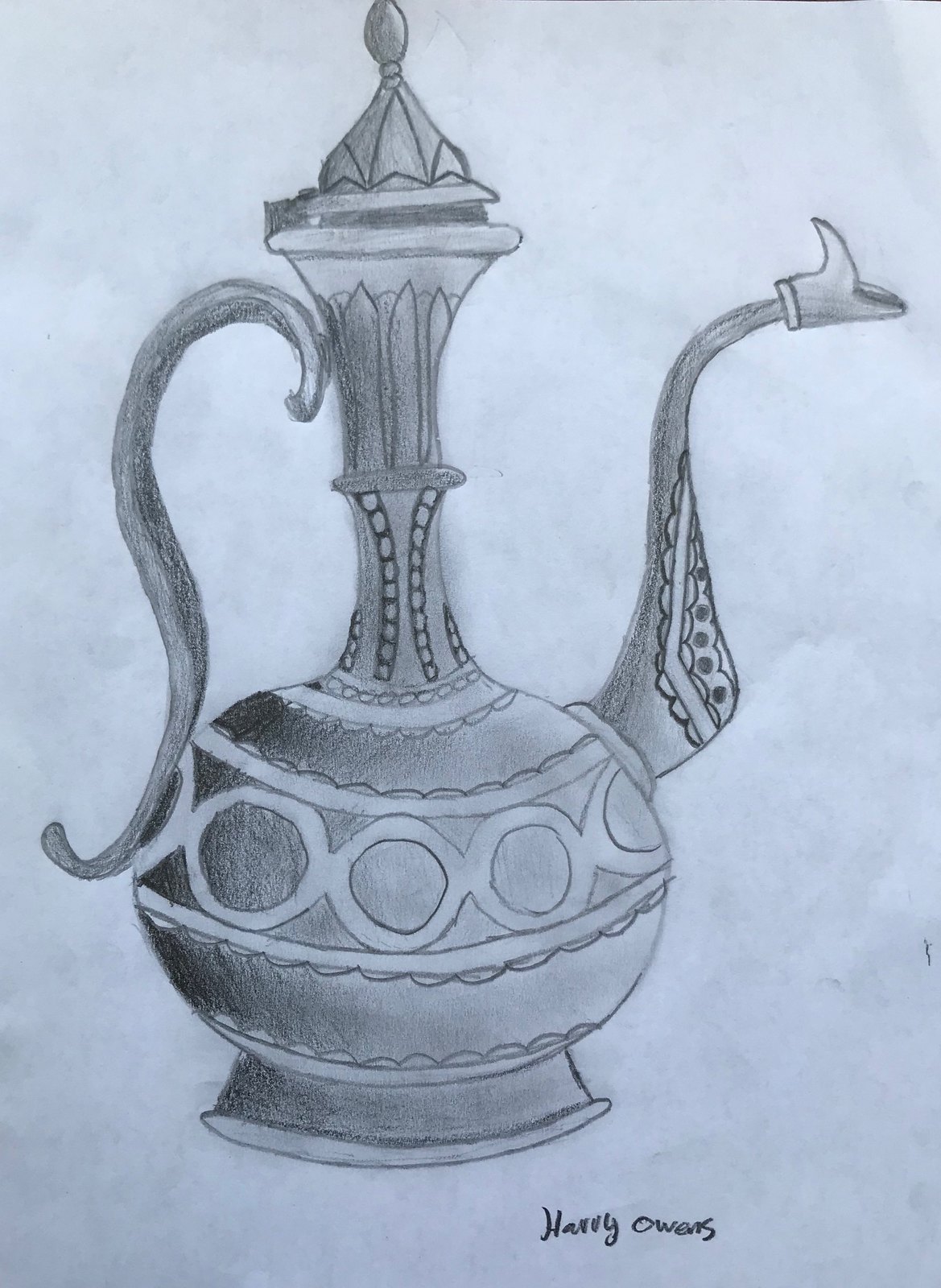This image showcases a highly detailed, elaborately shaded sketch of a tea kettle, possibly a Turkish teapot, drawn in gray and white tones. The tea kettle, centrally positioned, features a long S-shaped handle, an elongated spout, a bulbous body, and a tall neck with a swivel-attached lid. The teapot is adorned with intricate designs on the base, body, spout, neck, and lid. The artist's signature, "Harry Owens," is neatly placed at the bottom right of the drawing, suggesting an intentional and thoughtful composition. The overall style indicates that the drawing could have been created either as a hobby or a school project, with attention to capturing the elaborate parts and subtle details of the teapot.